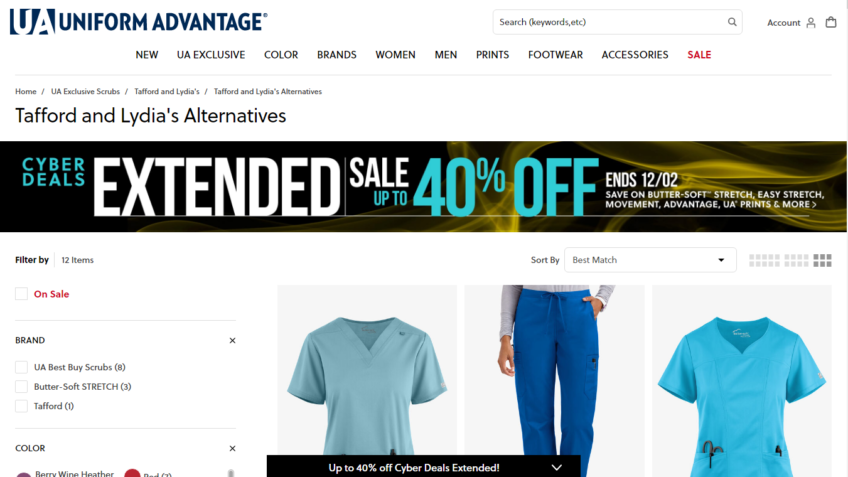The image is a screenshot of the Uniform Advantage website. At the top left corner, there is a red rectangle containing "UA" in a blue box, followed by the text "Uniform Advantage" with a registered trademark symbol (®) next to it. To the right, there is a search bar with the placeholder text "Search keywords," accompanied by a magnifying glass icon. Adjacent to the search bar, there are icons for account management (a person icon) and shopping (a shopping bag icon).

Beneath the header, there is a navigation menu with the following options listed from left to right: "New," "UA Exclusive," "Color," "Brands," "Women," "Men," "Prints," "Footwear," "Accessories," and "Sale" (the word "Sale" is in red font). A separating line below the menu leads to the next section, which prominently mentions "Taffert and Lydia’s Alternatives."

A large banner below advertises "Cyber Deals Extended" with a sale of up to 40% off, ending on 12.02, followed by additional sale information. On the left side, there is a filtering option labeled "Filter By," with a separating line underneath and a notice of "12 items" available. The "On Sale" section is highlighted in red, followed by a "Brand" section with three selectable options.

On the right side of the image, there are two displayed shirts, both in shades of blue and with V-neck designs, with what appears to be a pair of blue scrub pants positioned between them.